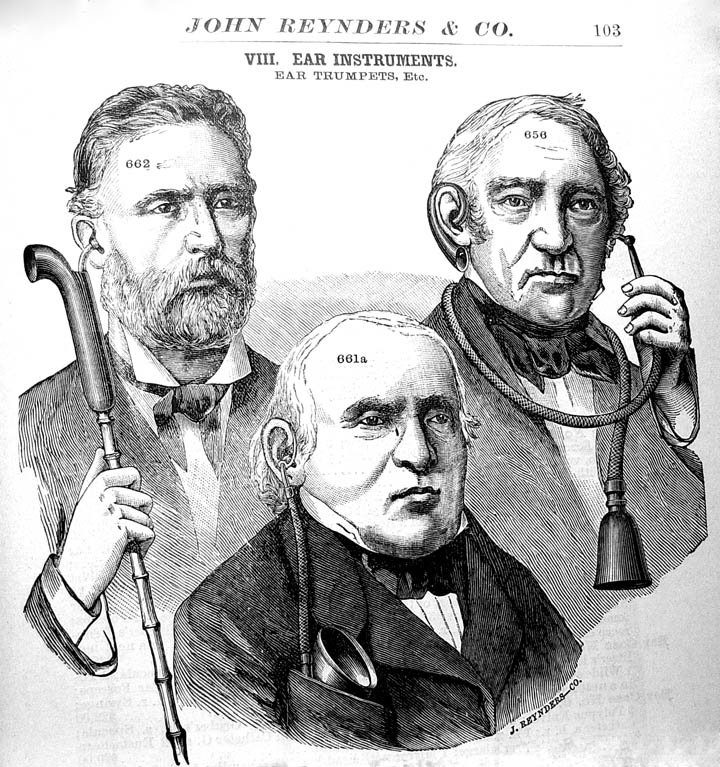This vintage pen-and-ink illustration, titled "John Randiers & Co., image 8, ear instruments, ear trumpets, etc.," is likely from a historical catalog or book. The square image features three older gentlemen drawn in grayscale on a white background, showcasing different types of ear trumpets—audiological aids from the past. 

In the center is a rotund gentleman with a receding hairline; his ear trumpet extends from his right ear into his coat pocket, where the larger listening device is concealed. This man, distinguished by his white hair, is dressed in a formal coat, tie, bow tie, and shirt. To his left is another gentleman with a full beard and a good head of hair. He is holding a sophisticated walking stick designed with a small piece that fits into his ear and a larger trumpet pointing towards the speaker. The gentleman on the far right demonstrates an early version of a hearing aid, resembling contemporary designs that curl around the ear. He handles a cord with a trumpet-shaped device at one end, which is placed into his right ear while looping around his neck. All three men are mid-chest up in the illustration, somberly displaying the devices without smiles, emphasizing the era's utilitarian approach to hearing aid design.